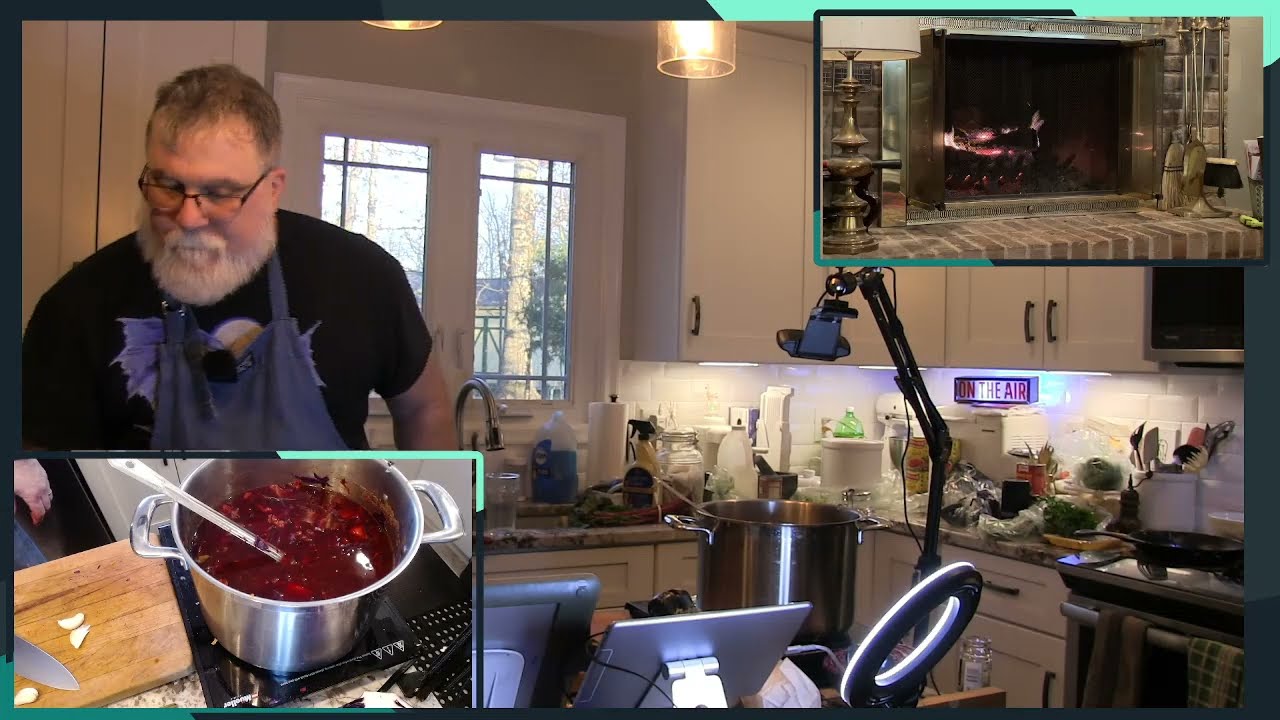In this cluttered kitchen, a man with a receding hairline and salt-and-pepper hair is cooking. He is wearing a black t-shirt with a design partially covered by a dark blue apron, eyeglasses with no lower frame, and has a thick white beard and mustache. The scene is busy with pots, pans, food, camera tripods, computer screens, and camera lights scattered around the counter. In the lower left corner of the image, a cutaway photo reveals a close-up of a large stainless steel pot on a burner, filled with red liquid and a silver spoon. To the top right, another cutaway photo shows a fireplace with brick sides and copper or brass accents. The kitchen cabinets are white, and there is a stand holding a cell phone positioned over the cooking area. An "On The Air" sign with "on the air" in red font and a black outline is visible in the far right center of the main image.